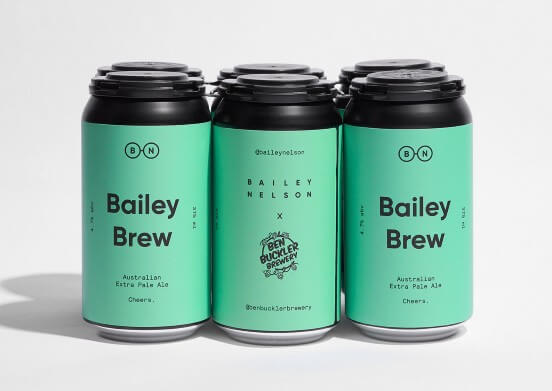This image showcases a six-pack of Bailey Brew, an Australian Extra Pale Ale, elegantly displayed against a white backdrop with a subtle shadow effect, likely designed for advertisement purposes. The cans, which appear to be aluminum with black reclosable tops, feature a primarily mint green label accented by black lettering.

The front-facing cans prominently display the name "Bailey Brew" in bold black caps, with "Australian Extra Pale Ale" beneath it, followed by the word "Cheers." The labels also include a logo featuring a circle with the letters "B-N," resembling glasses without ear pieces, situated on either side of the label's top. The sides of the cans additionally mention "Bailey Nelson" and "Ben Buckler Brewery," with a website or social media handle, though it is difficult to read. The cans' arrangement shows the design and branding from various angles, ensuring the brand and beer type are clearly visible.

Captured in detailed focus, this image genuinely portrays Bailey Brew as a sophisticated and inviting product, highlighting the sleek, modern design and brand identity of this microbrew.